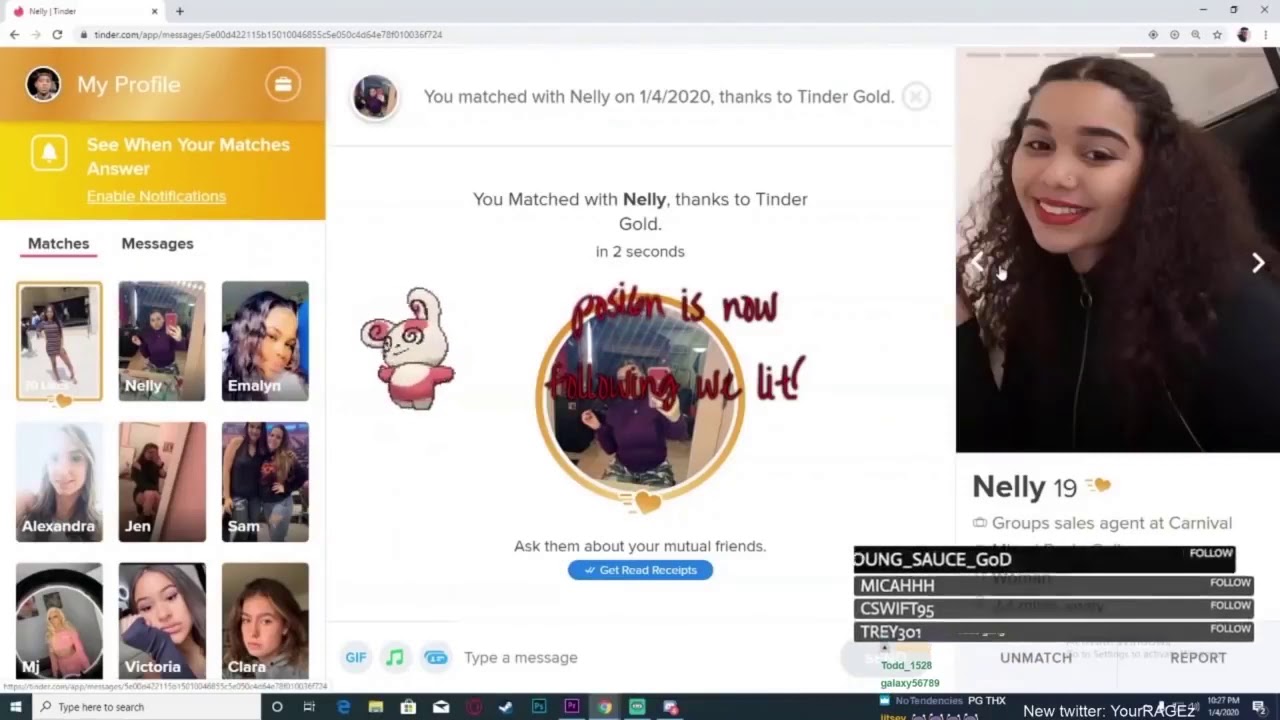The image is a rectangular interface, predominantly white with a gray band at the top. On the far left side, there are two orange icons. The first, a darker orange rectangle, reads "My Profile," while the lighter orange rectangle below it states, "See when your matches answer, enable notifications."

Below these icons, the section titled "Matches" is written in black letters with a red underline. This is followed by "Messages" and nine profile photos of different young women, suggesting it is a dating website interface. The names and pictures visible include Nellie, Emmaline, Alexandra, Jen, Sam, MJ, Victoria, and Clara, showcasing a diverse group with varying skin tones and hair colors.

At the center of the interface, the user's profile picture is displayed along with text indicating they matched with Nellie on January 4, 2020, thanks to Tinder Gold. Below this, another match notification with Nellie is shown. A gray line separates these sections. There is a small bunny rabbit icon and circled text that appears partially obscured but suggests a statement about meeting. Underneath this is a prompt to "Ask them about your mutual friends," and further down, there is a message about getting something, shown with a white checkmark that is too small to discern.

Icons for sending gifts, music, and typing messages are also visible.

On the right side of the screen, there is a large photo of Nellie, a young woman with mixed-race appearance, curly black hair, light brown skin, and red lipstick. Her name, age (19), and username "Young Sauce God" are displayed. Beneath this, several usernames—Micah, CSwift95, and Trey301—are listed inside black rectangles with "Follow" buttons in white letters.